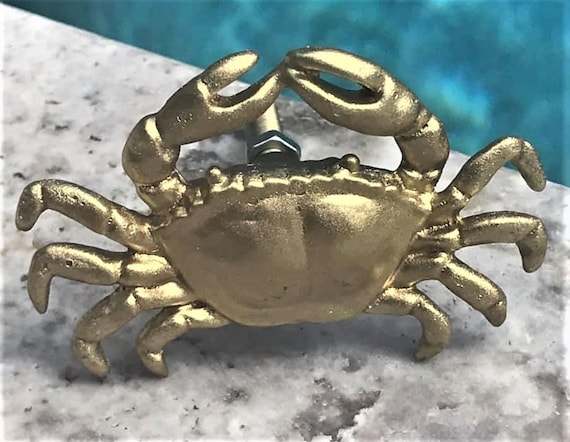The photograph depicts a shiny, gold-painted metal crab standing upright on a white and gray granite countertop, with a dark blue background. The crab is intricately designed with two eyes, eight legs, and two claws raised up and touching above its head. Its surface is slightly rough, adding texture to its metallic sheen. The crab appears to be part of a fixture, possibly a hardware component or a decorative piece, with a metal pipe and a nut extending from its bottom, suggesting it might function as a faucet handle, cabinet fixture, or some sort of spigot. The crab's detailed features and its golden color make it a notable and eye-catching item.